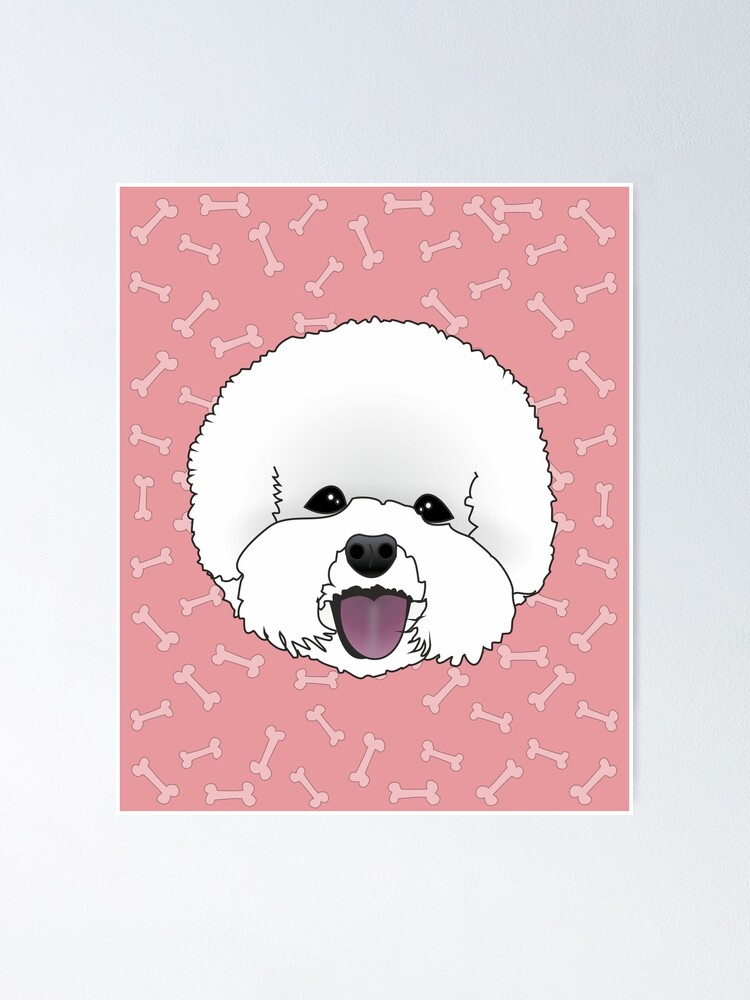The image features a prominently placed piece of art on a white wall. Central to this art piece is the face of a small, white dog, resembling a fluffy toy poodle or a tiny terrier, characterized by its fuzzy hair, big black eyes, black nose, and a slightly protruding tongue that carries a pinkish-red hue. The dog's face, including its fluffy ears, is the sole focus with no body shown, and it has a distinctive mustache-like fur around its mouth. The background of the poster is a light pinkish-peach color adorned with a repetitive pattern of cartoon dog bones. These bones have a lighter pinkish-peach color and are outlined in black, creating a visually engaging pattern across the background. The artwork is rendered in a simplistic yet detailed manner with complete outlines surrounding the dog, giving it a minimalist yet defined appearance. The overall presentation suggests it could be computer-generated to resemble a drawing or a 3D effect, enhancing the playful and whimsical nature of the depicted scene.